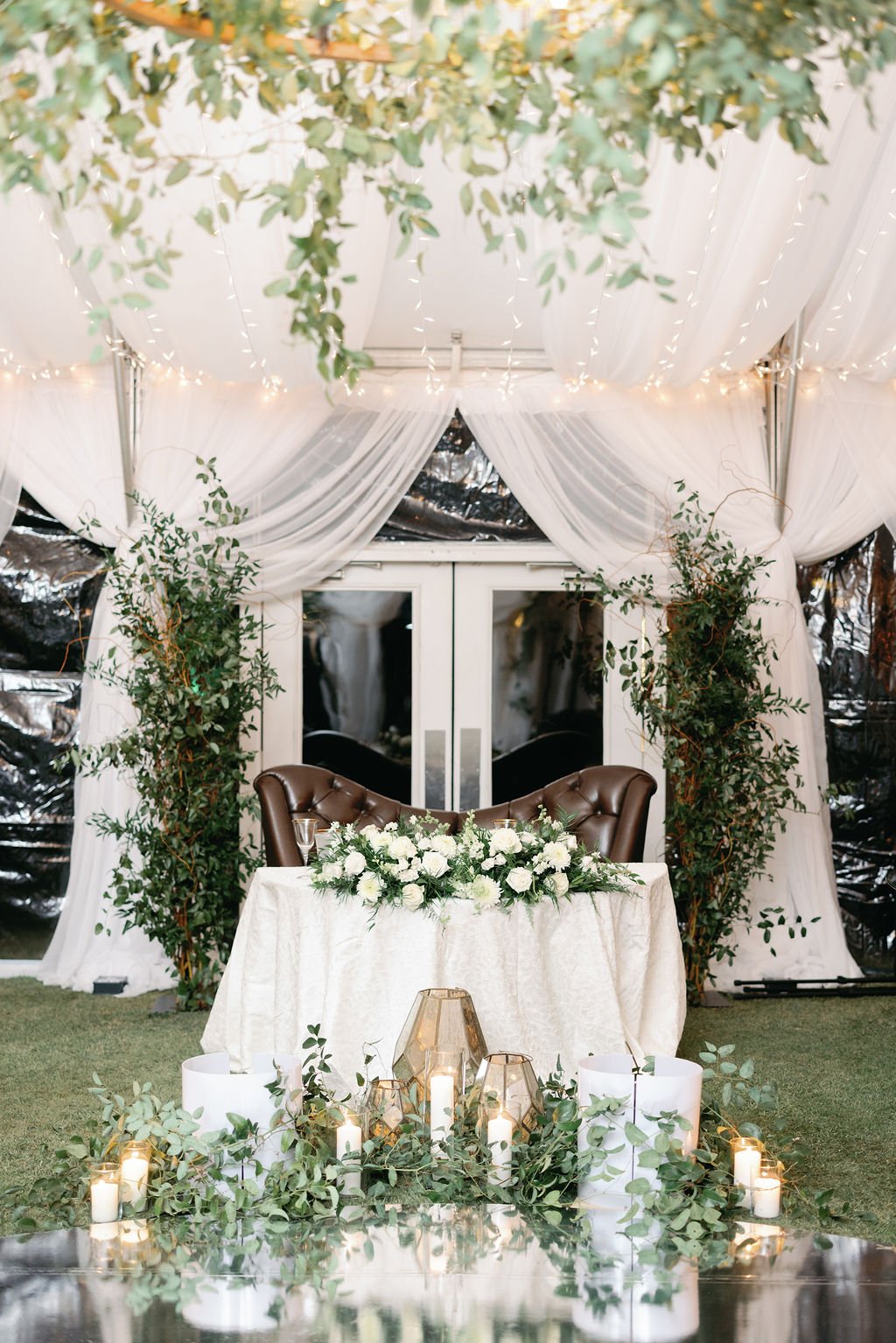In the image, an outdoor wedding ceremony area is beautifully illuminated and well-decorated. The centerpiece is a double door with blackish glass panes, adorned with draped white curtains cascading down and anchored up into the overhanging trees with string lights strung across the top. A wooden chair for two sits invitingly in front of the door, positioned behind a white table covered in white linen and a lavish bouquet of white roses. In front of this table stands another arrangement, a table filled with a variety of lit candles in different shapes and sizes, surrounded by an abundance of foliage and floral arrangements. The scene is framed by a wooden fence and punctuated by the lush greenery of nearby trees and branches, creating an elegant and enchanting setting for the bride and groom.